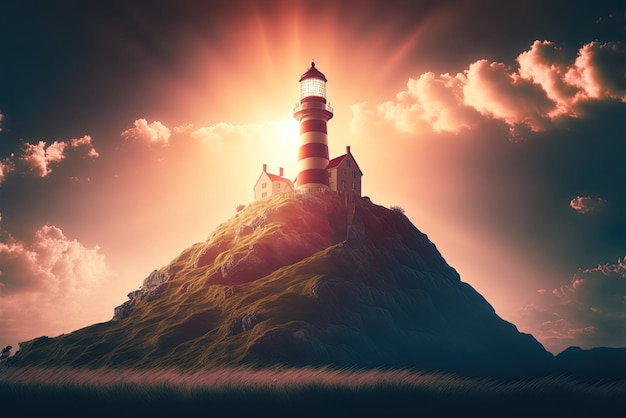This image, possibly a painting or AI-generated, features a striking lighthouse positioned majestically atop a large, grassy hill that transitions into areas of long, tan grass at the base. The lighthouse, adorned with red and white candy-cane stripes and a red top, stands prominently between two small houses with white walls and red roofs. The scene is set against an evening sky filled with clouds, where the sun emits a brilliant glow from behind the lighthouse, almost illuminating the entire sky as if it were daytime. The dramatic lighting emphasizes the lighthouse's vibrant presence, making it a focal point that illuminates the surrounding landscape. The rocky hill beneath the lighthouse slopes downwards, flanked by undulating green hills, creating a picturesque and serene environment. The intricate details of the red catwalk and the sun's reflection enhance the overall majesty of this stunning portrayal.